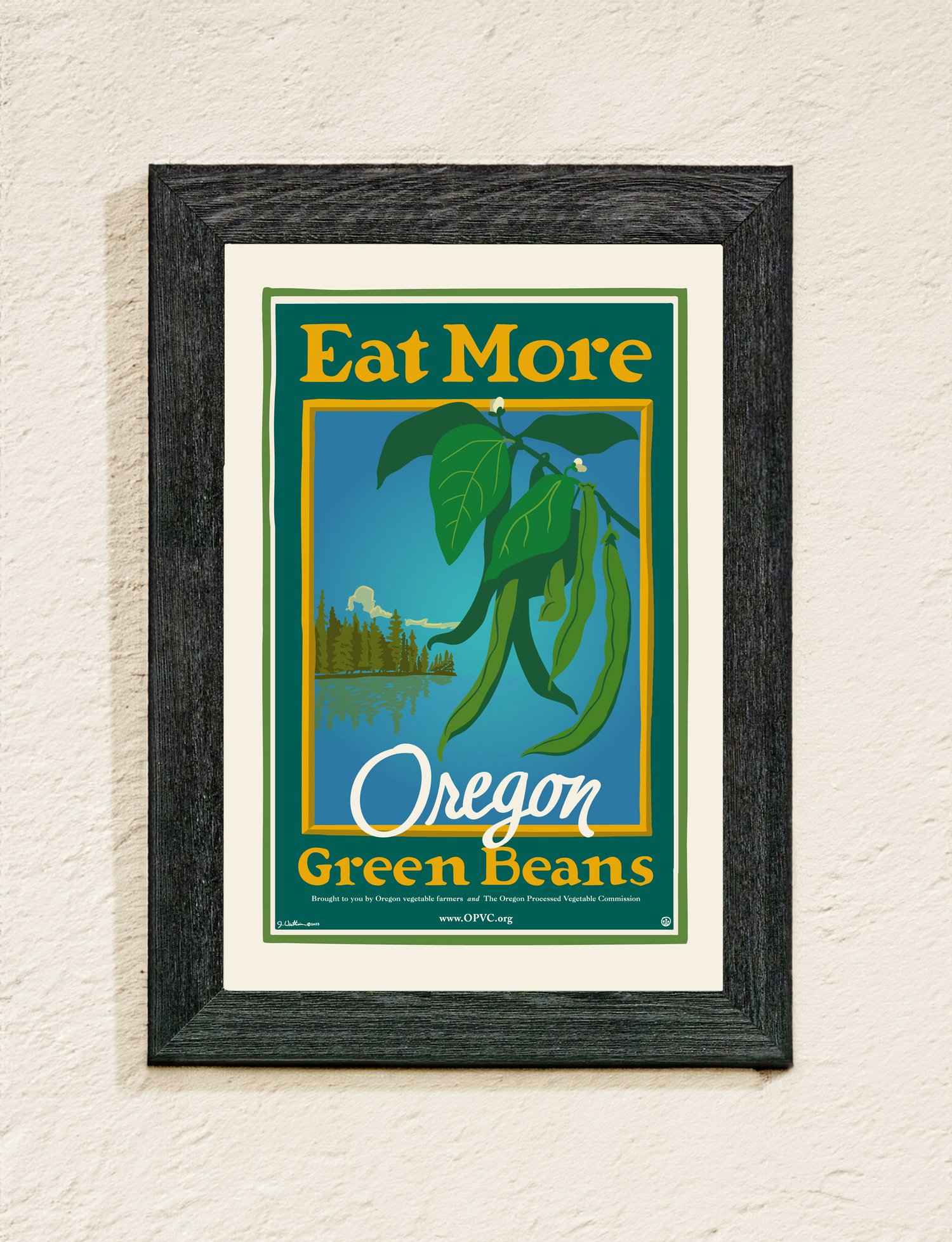The image features an old advertisement poster for Oregon green beans, prominently displayed within a walnut wood-grain frame that appears black. The central message reads "Eat More" in yellow at the top, and "Oregon Green Beans" in matching yellow text at the bottom. The main illustration showcases green beans on the vine, with lush leaves above and a serene backdrop of pine trees by a lakeside under white clouds. Beyond the image, a multi-layered border ensues: a thin white line, a surrounding green line, and a larger white matting, all enclosed by the black wooden frame. Additionally, the poster includes a green banner with the website "www.opvc.org". The background of the setting reveals a white plaster-like wall, accentuating the framed advertisement.